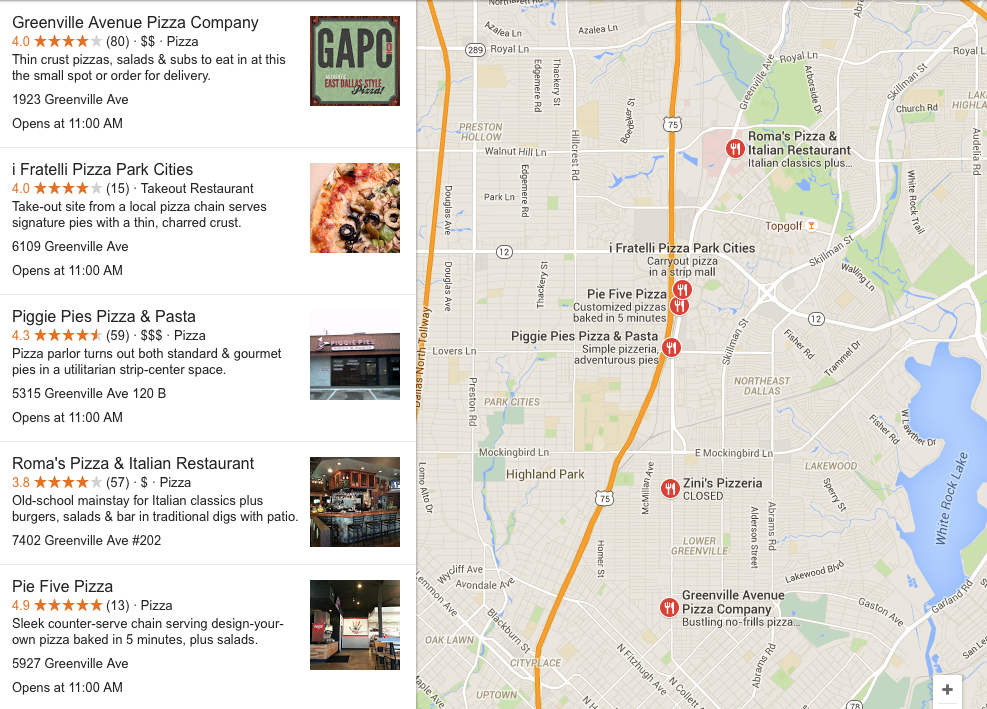The image is a screenshot of a website displaying a search result page for pizza restaurants. The left side features a list of five different pizza establishments, each on a white background with black text, detailing various aspects of the restaurants. The first one is "Greenville Avenue Pizza Company," which includes a logo with green, black, and red elements, the opening hours, and customer ratings displayed in orange stars. Another entry is "Airfragili Pizza Park Cities," showing a 4.0 rating, takeout options, operating hours, and the venue's address. Each restaurant listing follows a similar format, providing an image of their offerings, ratings, and contact details. On the right side of the image is a map, pinpointing the locations of these restaurants, aiding users in finding their desired dining spot visually.